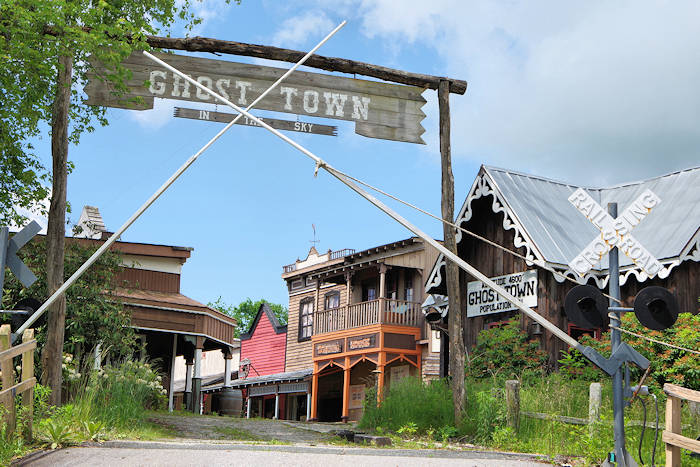The image depicts the entrance to a Western-style ghost town, marked prominently by a wooden sign suspended between two poles that reads "Ghost Town in the Sky." In the foreground, white railroad crossing arms are visible, adding to the rustic charm of the scene. A series of stylized Western buildings line the background, beginning with a structure on the right that displays an inscription about an altitude of 4,600 feet, the name "Ghost Town," and a population figure obscured by the crossing arms, likely indicating a small population in double or triple digits. Adjacent to this, a two-story building with a balcony stands proudly, its exterior painted in varying shades of brown and orange. Other Western-themed buildings trail off into the distance, contributing to the quaint, nostalgic atmosphere of the ghost town.